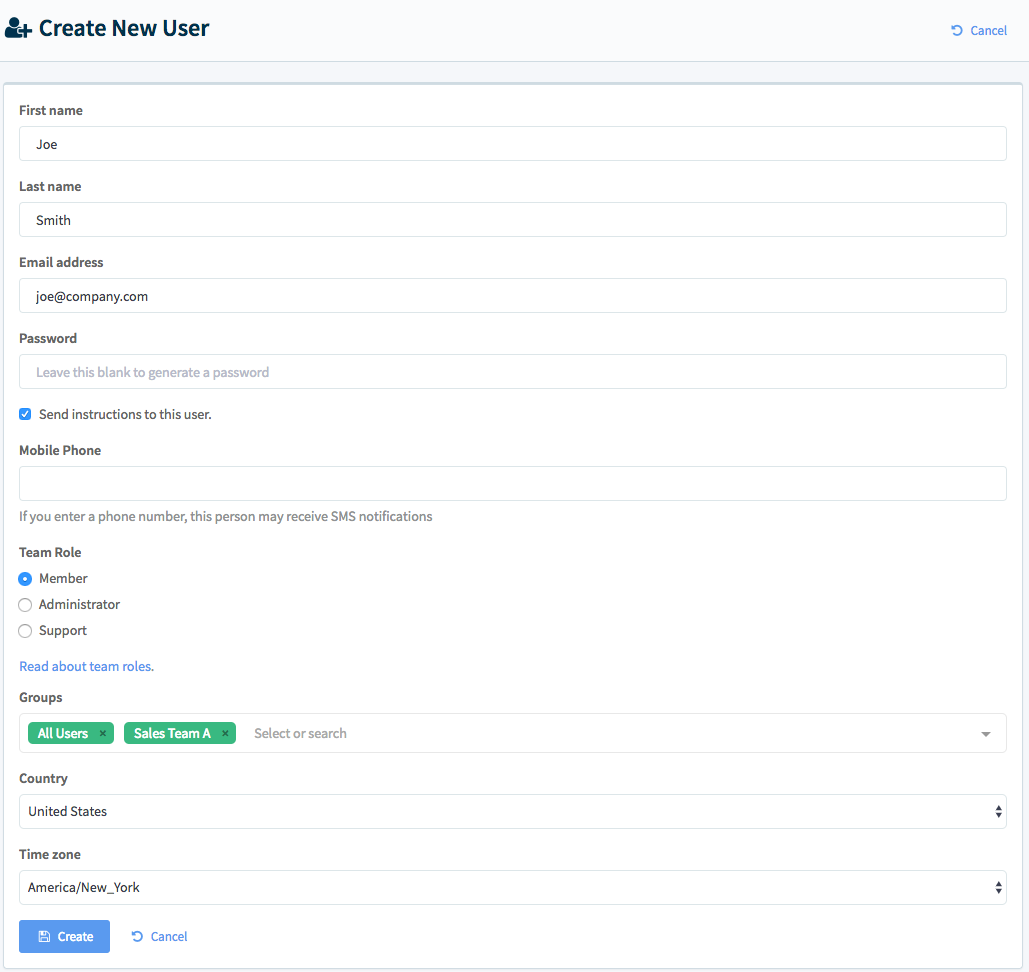In this image, you can see a user registration screen with a clean, white background. At the top left corner, the heading reads "Create New User," accompanied by a small "Cancel" option in blue on the right. Below the heading are several input fields and options. The first field is labeled "First Name" and contains the name "Joe." Next is the "Last Name" field with "Smith" entered. The "Email Address" field is filled in with "joe@company.com," while the "Password" field remains empty.

Beneath these fields, there is a checkbox labeled "Send instructions to this user," which is checked and displayed with a blue square and a checkmark. Following this is the "Mobile Phone" field, which is currently empty. 

The "Team Role" section offers three options—"Member," "Administrator," and "Support." The "Member" option is selected. Right below this section, there is a link in blue text that says "Read about team roles."

Next is the "Groups" category, showing options for "All Users" and "Sales Team A," with "Sales Team A" highlighted in green. Following that, the "Country" field indicates "United States," and the "Time Zone" field displays "America/New York."

At the bottom of the form, there are two buttons side by side. The left button is a blue "Create" button, while the right button is white with "Cancel" written in blue text.